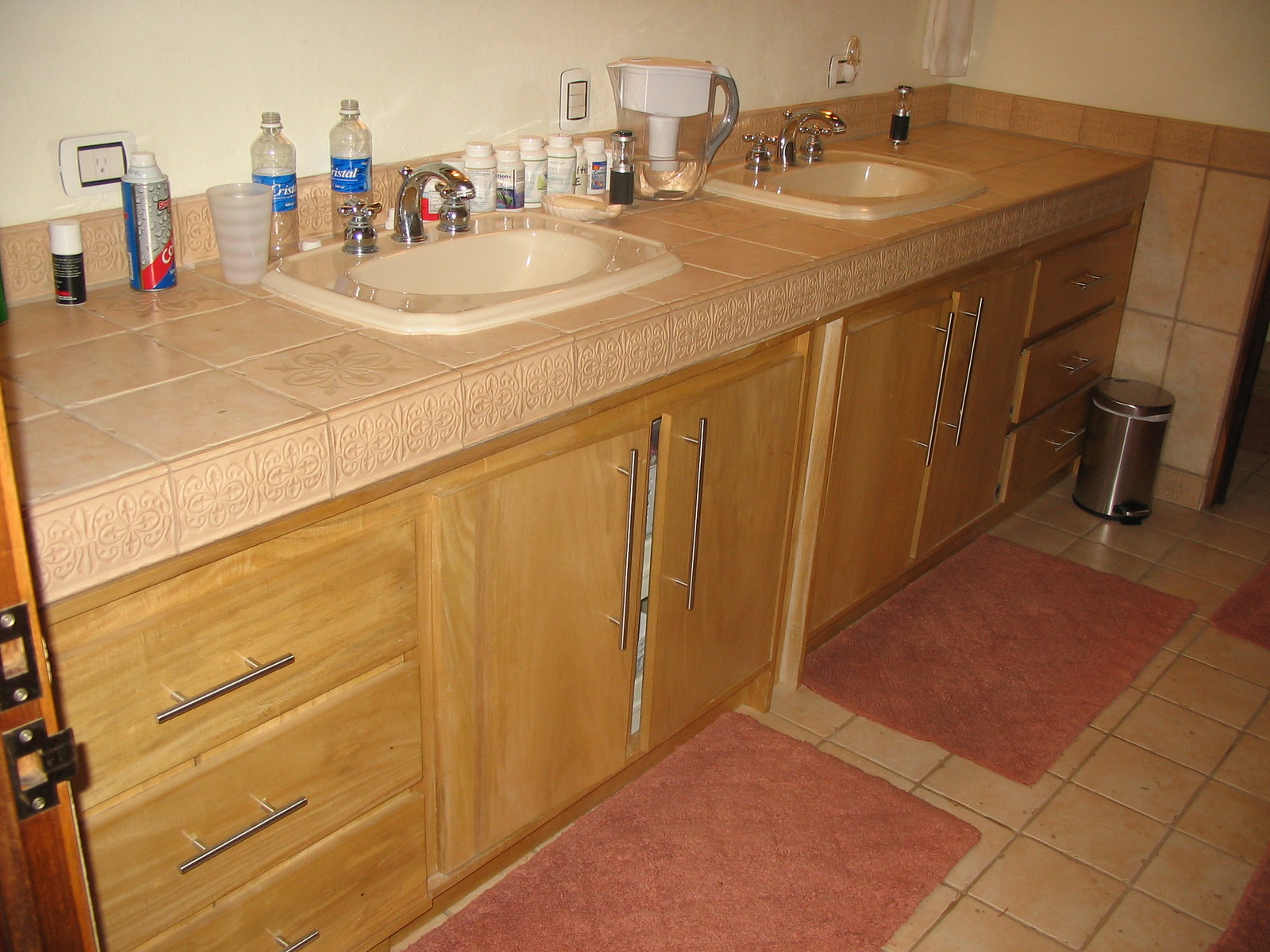The image depicts a neatly organized double sink area in a well-maintained restroom. Each sink, located on the right and left, is made of pristine white porcelain and is equipped with stainless steel faucets and handles. The sinks stand on a countertop made of white stone tiles, providing a clean and sophisticated look. Below the countertop are wooden cabinets featuring a combination of pull-out drawers and swing-open doors, offering ample storage space.

In front of each sink, there are light red rugs that add a touch of warmth and comfort against the floor, which is tiled with square stone tiles that match the countertop in quality and style. Positioned in the upper right center of the photo is a small stainless steel trash can, blending in unobtrusively with the overall decor.

On the countertop behind the sinks, various personal items are neatly arranged. These include a bottle of shaving cream, a couple of bottles of water, and several white bottles that seem to contain vitamins and supplements. Among these items is a glass water jug equipped with a water purifier, indicating a commitment to clean, filtered water in the household. Overall, the image presents a functional and aesthetically pleasing double sink area that reflects good organization and attention to hygiene.